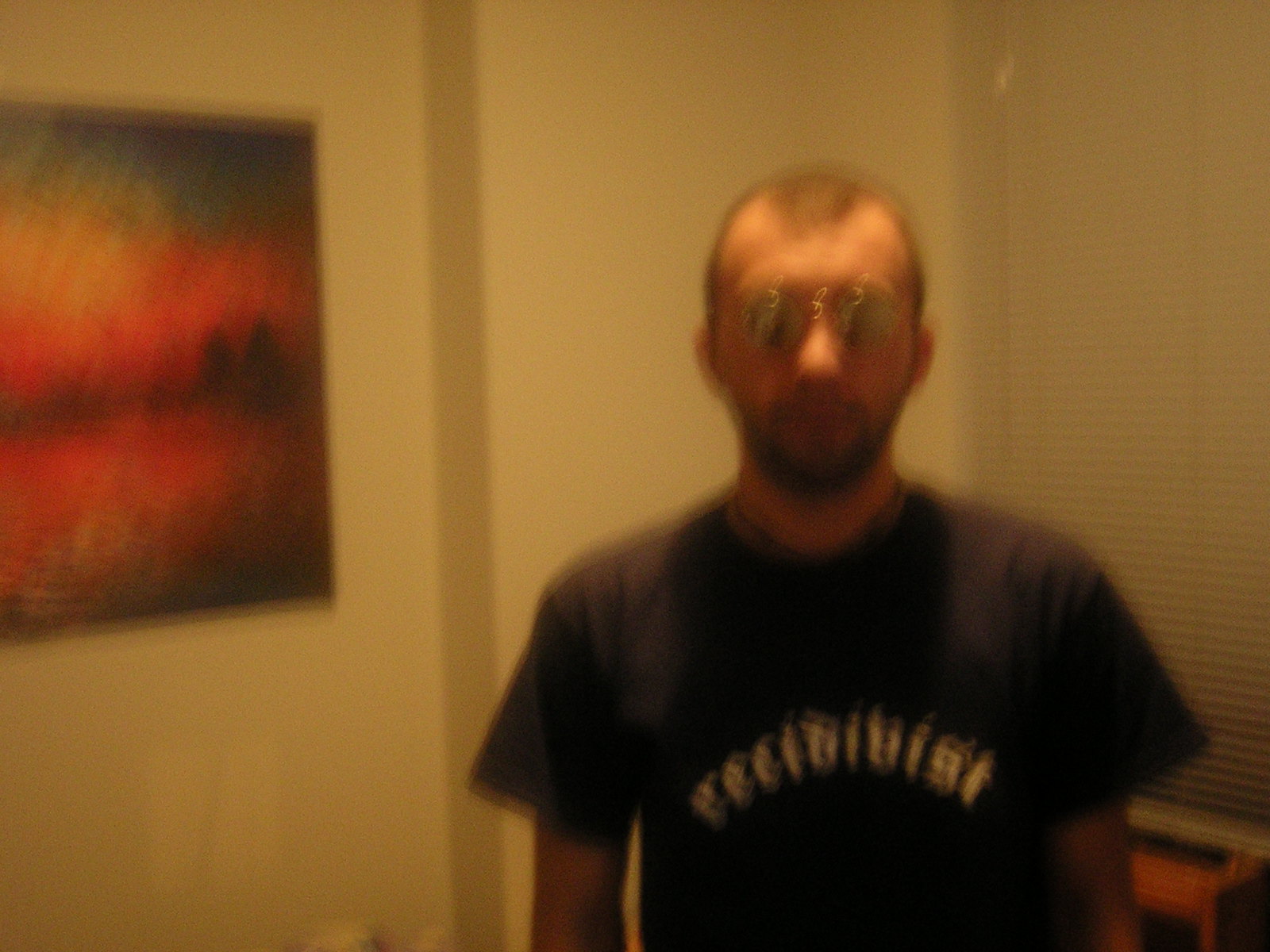In this slightly blurry photograph, a man stands towards the middle-right section of a room. The motion blur suggests the camera was in motion as the photo was taken, rendering the scene a bit fuzzy. The man, who is Caucasian and sports an almost shaved head, wears a dark t-shirt with illegible white text. He has round sunglasses and short facial hair. The background features vertical blinds covering a window and a plain wall. To the left of the man, a painting depicting a serene sunset over a lake adds a splash of color to the otherwise simple setting.